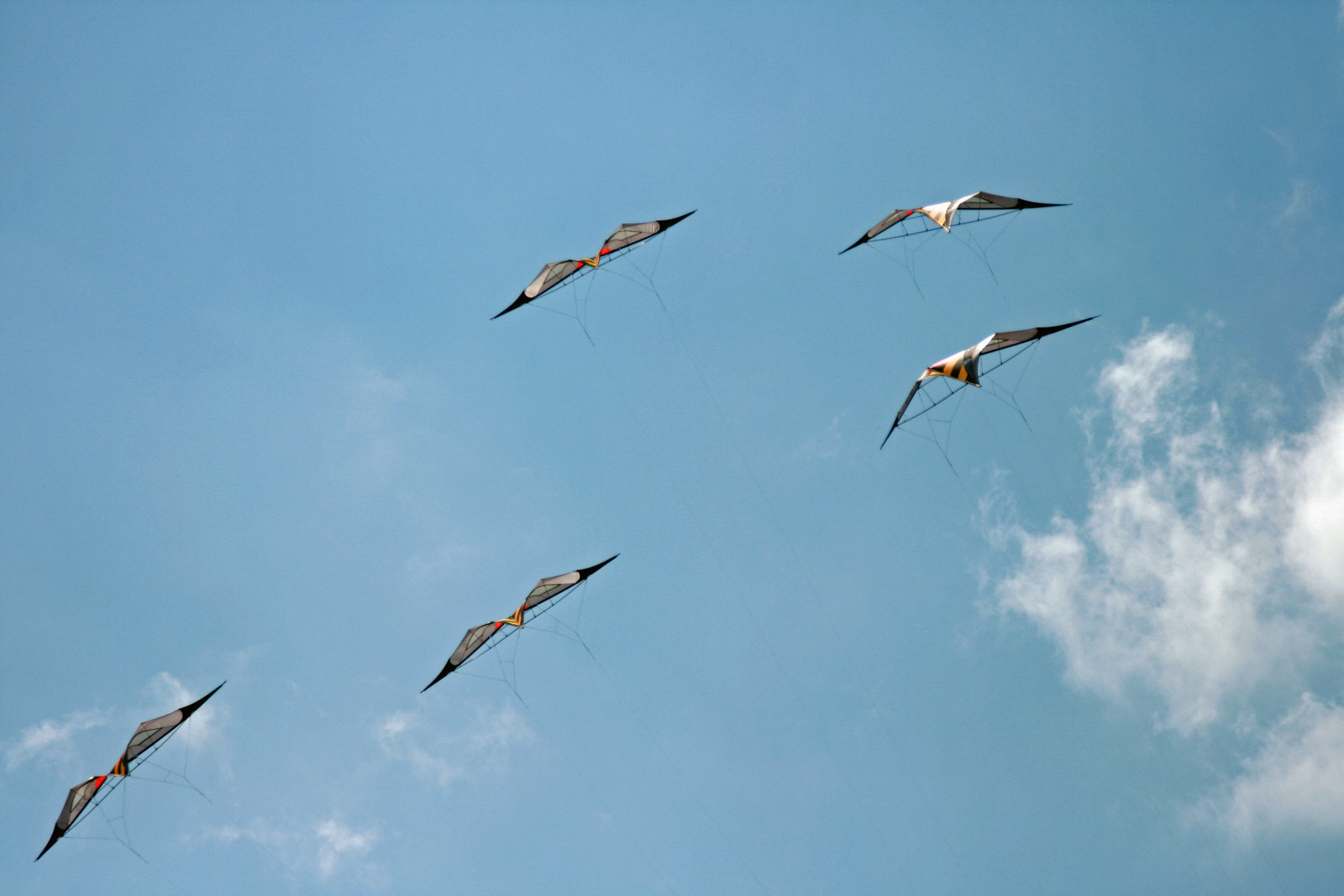In this photograph, five kites soar gracefully in a bright, light blue sky adorned with minimal cloud cover. The sky is predominantly clear, with a few wisps of clouds in the bottom-left and some denser clouds on the far right. The kites, all facing the same direction, are designed to resemble birds with their wings spread out. Each kite features a triangular front portion that arches to each side, creating a swooped-down wing shape. The wings are tipped in black and have an orange beak-like protrusion at the front with black and white accents. Faintly visible, almost transparent strings connect the kites, descending in two lines from each one. The kites are arranged with one in the lower left corner, another slightly to its right and lower, one above the second kite toward the right, and two more to the right below the third kite, forming a visually appealing pattern against the serene sky backdrop.